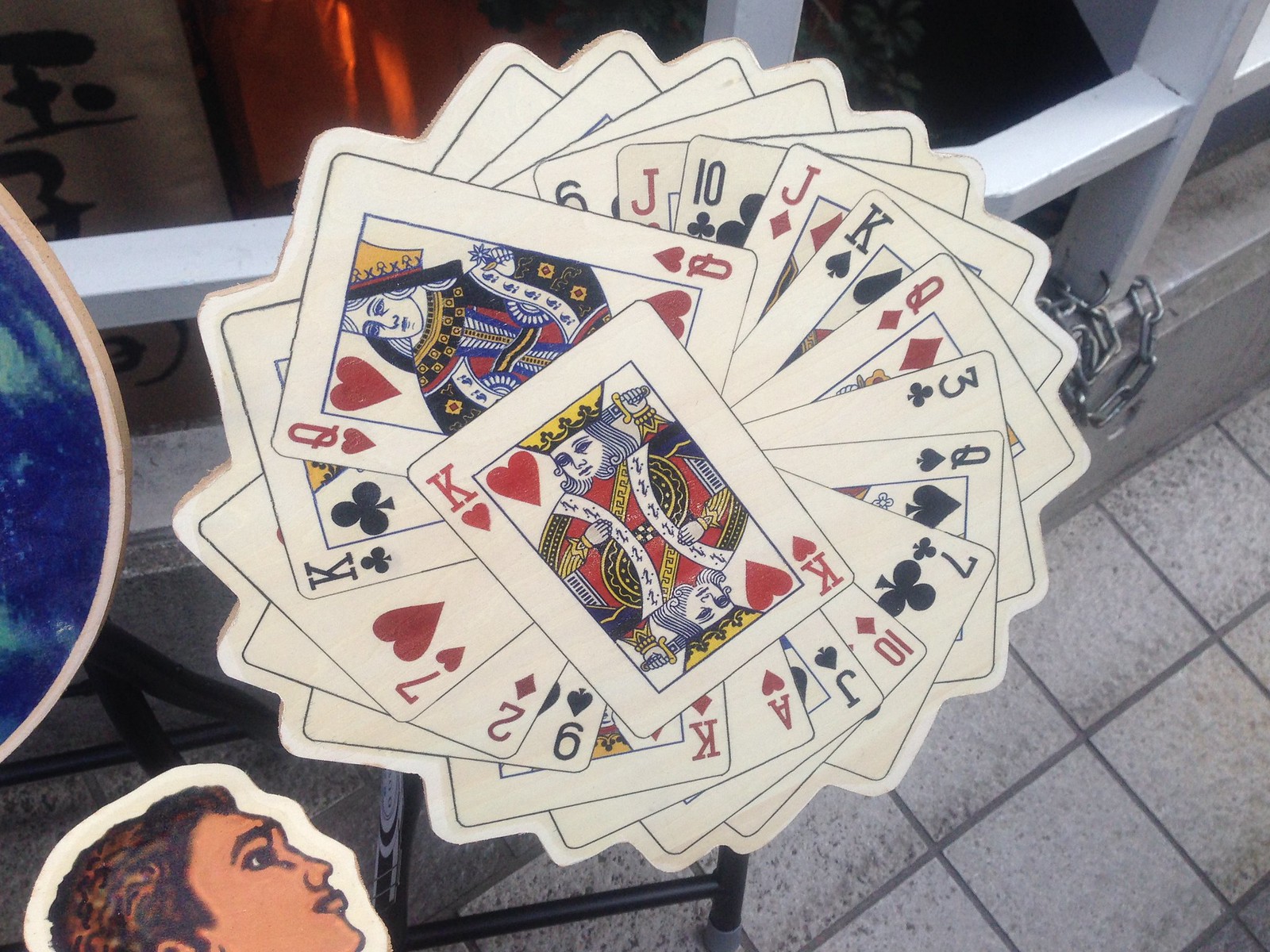The photograph captures a gray square tile floor with a variety of objects and details on the left side. Dominating the left side is a partially visible wooden sign, characterized by its rounded shape and brown hue, adorned with blue and light green colors reminiscent of a globe or sea. The wooden sign stands on a black base, possibly supported by metal pipes. Nearby, in the far left corner, there is a fabric sign featuring foreign script written vertically in black, adjacent to a piece of reddish-orange fabric whose purpose is unclear.

The wooden sign appears to be resting against a metal canopy or balcony structure. Positioned next to this is another notable sign, depicting a circular arrangement of playing cards, including the King and Queen of Hearts, and various suits such as spades and clubs. This sign leans on a black metal stand and another part of the light gray balcony structure, which also houses a metal cane protruding from one of its poles.

In the bottom left corner of the image, there's another partially visible wooden sign with a white background. This sign cuts off at a person's chin, leaving most of their face and ears obscured. The overall composition presents a rich assortment of textures, colors, and objects, creating a vivid and complex scene.